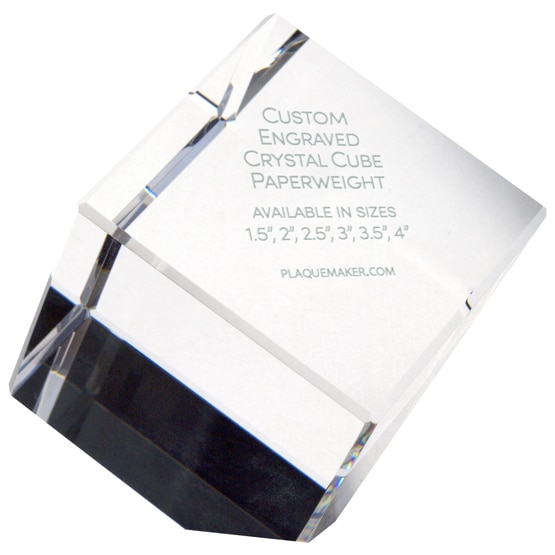The image features a tilted, crystal glass paperweight suspended mid-air at the center of the photograph. The paperweight, with a diamond-like, or more precisely, rhombus-like shape, is divided into two distinct sections: a clear, crystalline top and a solid black bottom. Engraved text at the upper, clear section of the paperweight reads "CUSTOM ENGRAVED CRYSTAL CUBE PAPERWEIGHT AVAILABLE IN SIZES 1.5", 2", 2.5", 3", 3.5", AND 4"." The text appears to be in capital letters and sports a simplistic design. Below this text, closer to the base in the black section, the URL "plaquemaker.com" is etched, likely indicating where the product can be purchased. The background of the image is stark white, suggesting a clean, office supplies or stationery context.